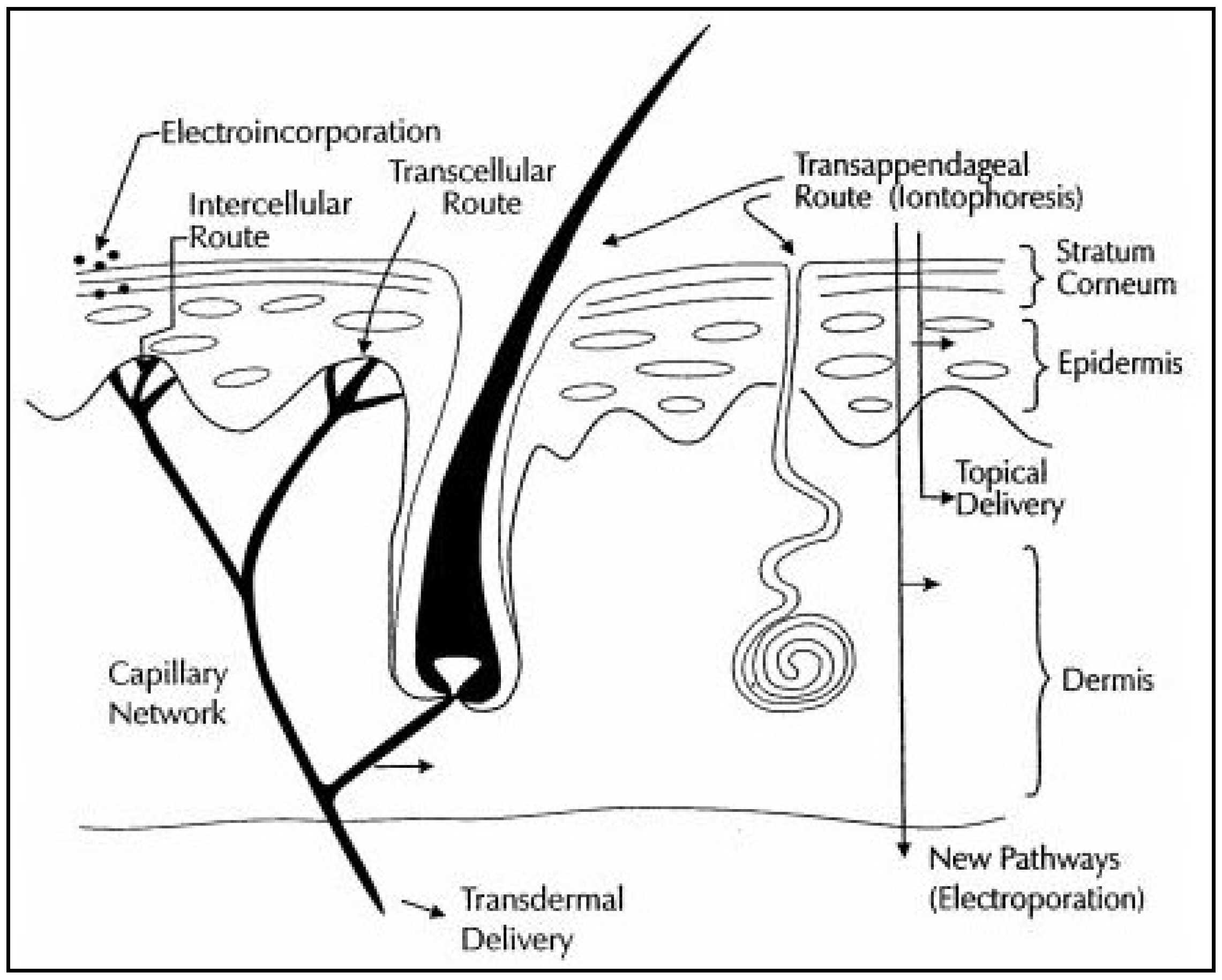This is a detailed, black-and-white textbook diagram that illustrates the different pathways of skin and hair growth in a scientific context. The diagram displays a cross-section of skin with various labeled components, including the Capillary Network, Stratum Corneum, Epidermis, and Dermis. Arrows indicate different routes and processes such as Electroin Corporation, Intercellular Route, Transcellular Route, Transappendageal Route, and Transdermal Delivery. Additionally, it shows pathways for Topical Delivery and highlights New Pathways Electroporation. In the diagram, the hair follicle is visible, extending from the root within the skin to the hair shaft outside. The image uses black text and drawings on a white background, with arrows guiding the viewer through the technical details, similar to what you would find in a clinical or technical textbook.